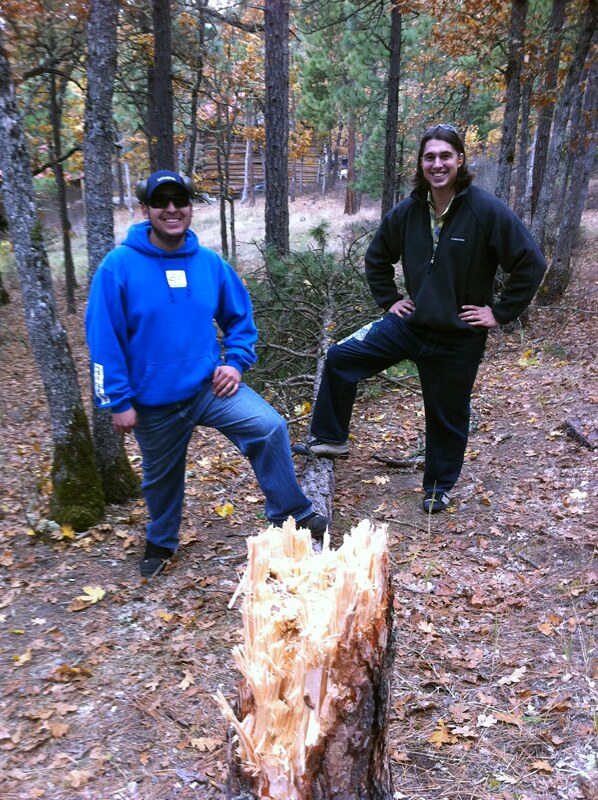In the heart of a lush, forested area, two young men are captured in a candid moment of triumph. The focal point of this outdoor photograph is a freshly snapped tree stump, emphasizing the raw edges where the tree has broken, with splintered shards pointing in every direction. Behind the stump lies the felled tree, and each man has one foot propped confidently on the massive trunk, their faces beaming with proud smiles.

To the left stands a man clad in a royal blue hoodie, jeans, and black sneakers. His left foot is positioned on the fallen tree, and his left hand rests on his thigh. He wears a dark blue baseball cap, and his eyes are concealed by sunglasses, which he wears over a set of headphones. His friend, slightly taller, stands on the right side, dressed in a dark jacket over a light green button-up shirt, dark blue pants, and black and beige shoes. His shoulder-length hair cascades around his smiling face, and a pair of sunglasses rest on the top of his head. 

Both men emanate satisfaction, likely having been the ones to bring down the tree they now pose with. A log cabin peeks through the trees in the background, further encapsulating the serene, verdant setting of their woodsy adventure.